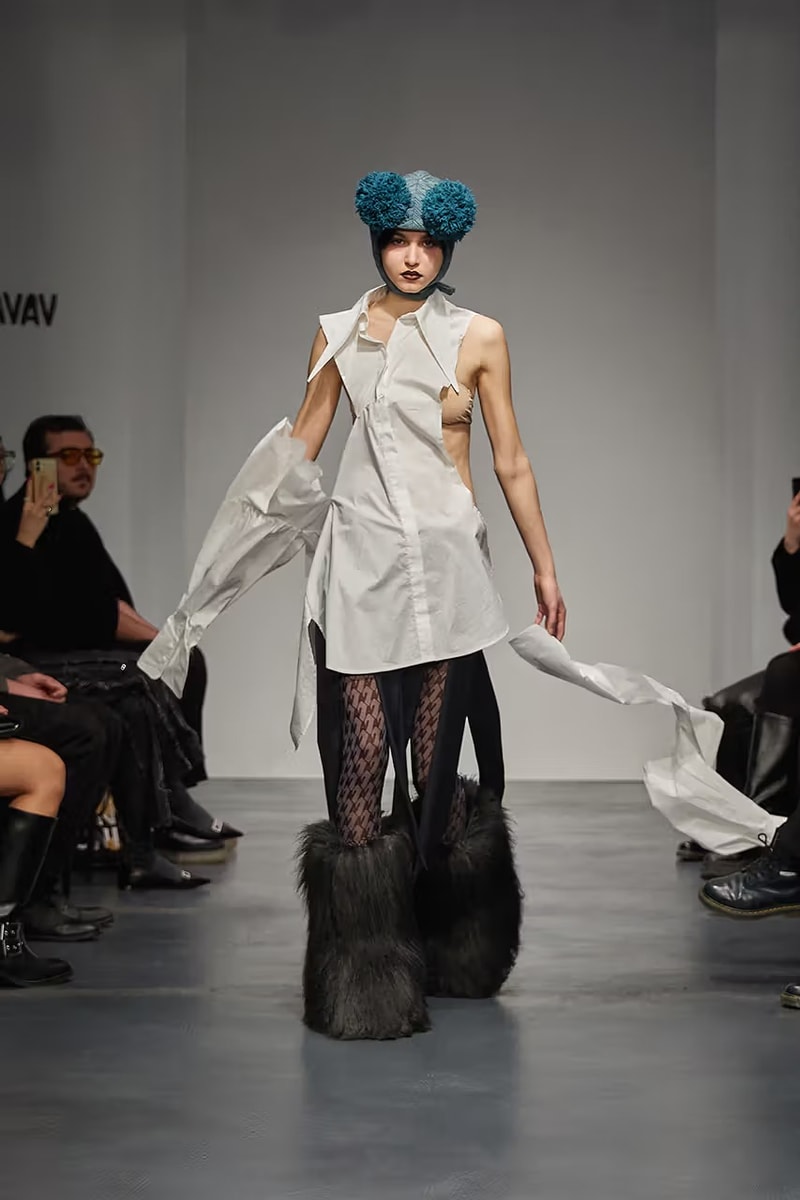The image is a highly detailed color photograph capturing a model walking directly towards the camera on a runway. She’s adorned in an intricate and unconventional outfit that features a striking blue hat with two enormous blue-green pom-poms prominently displayed in the front, secured under her chin with black straps. Her expression is serious, accentuated by bold red lipstick. The model's white, long-sleeved button-up shirt is dramatically shredded, leaving her sides and arms exposed. Her right arm is partially covered by a tattered sleeve up to the elbow, while her left arm is completely bare. She complements this attire with black fishnet stockings and enormous, shaggy boots resembling mammoth feet, extending almost to her knees. The runway floor is gray, and she is flanked by an audience dressed in black, observing her meticulously. The backdrop is primarily white with some text that is partially legible, revealing the letters "V, A, V" in black above the audience on the left side.